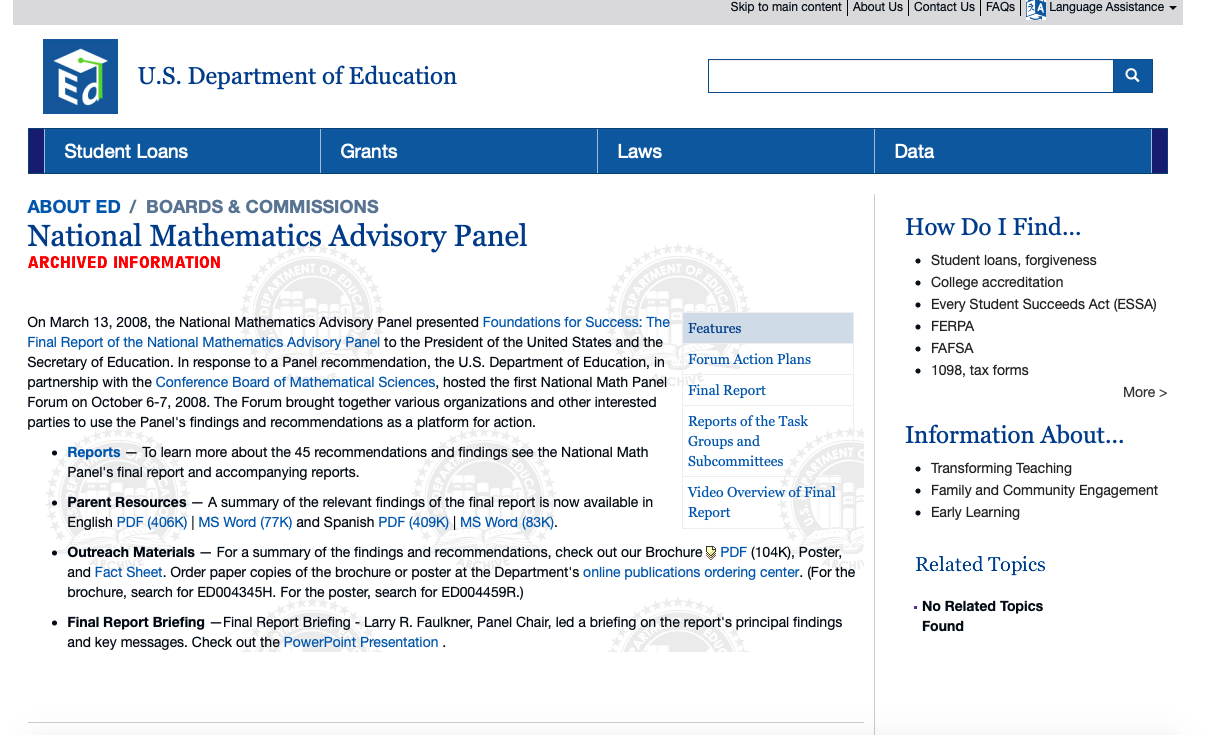The image depicts a webpage from the US Department of Education, prominently marked in the upper left-hand corner. The page boasts a distinctive logo featuring a capital "E" and "D" inside a box, with the "D"'s outer edge and a tassel extending over the box edge in lime green, resembling a graduation cap.

At the top, a gray navigation bar provides quick links labeled "Skip to main content," "About Us," "Contact Us," "FAQs," and "Language Assistance." Below this, a blue bar offers more specific links including "Student Loans," "Grants," "Laws," and "Data," followed by "About ED" and "Boards and Commissions."

The main content section highlights the National Mathematics Advisory Panel, marking archived information in red. It describes a historical note dated March 13, 2008, when the National Mathematics Advisory Panel Board presented "Foundations for Success." The text features both red and black letters, with certain clickable blue hyperlinks directing to reports, parental resources, outreach materials, and a final report briefing. 

Behind this writing, faint seals add a watermark-like layer to the design. Additional content boxes outline featured elements like forum action plans, task group and subcommittee reports, and a video overview of the final report. 

On the right side of the page, a section titled "How do I find" provides further navigation assistance and related topics, enhancing the user's ability to locate specific information.